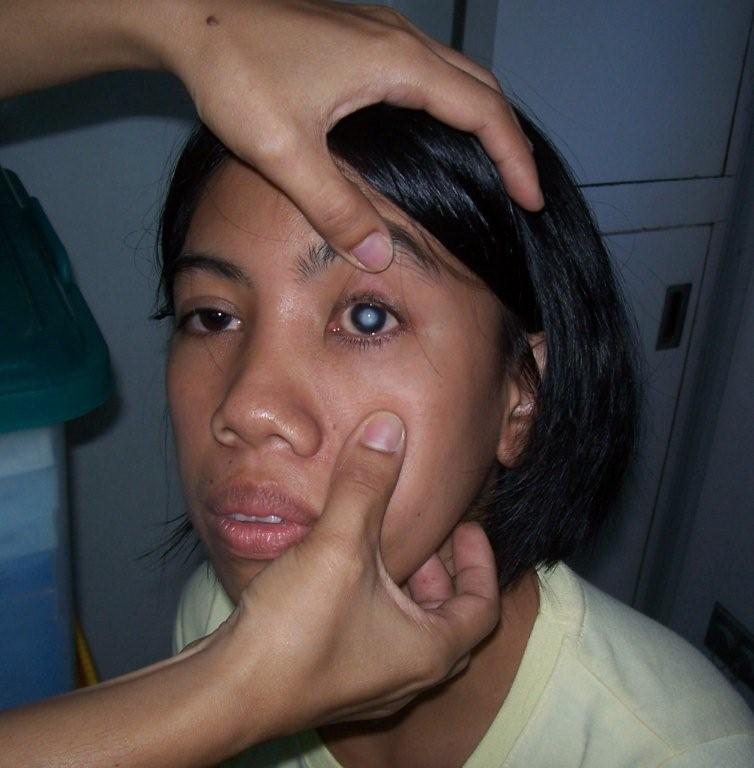In the image, a woman with shoulder-length dark brown hair and a tan complexion is seated in a white room. She wears a yellowish shirt and has a few distinct freckles: two above her lip and one on her cheek next to her nose. Her expression is blank, and her gaze is slightly to the side of the camera. 

A pair of hands, presumably a man's, are holding her right eye open using their thumbs, placed above and below the eye, stretching it wide. This eye shows a large, white discoloration in the center, some redness, and appears slightly swollen, creating an unsettling contrast with her normal dark brown left eye.

Behind her, there's a white cabinet with a visible handle, and to the left side of the image, a plastic storage bin with a green top, containing various small boxes, is partially visible.